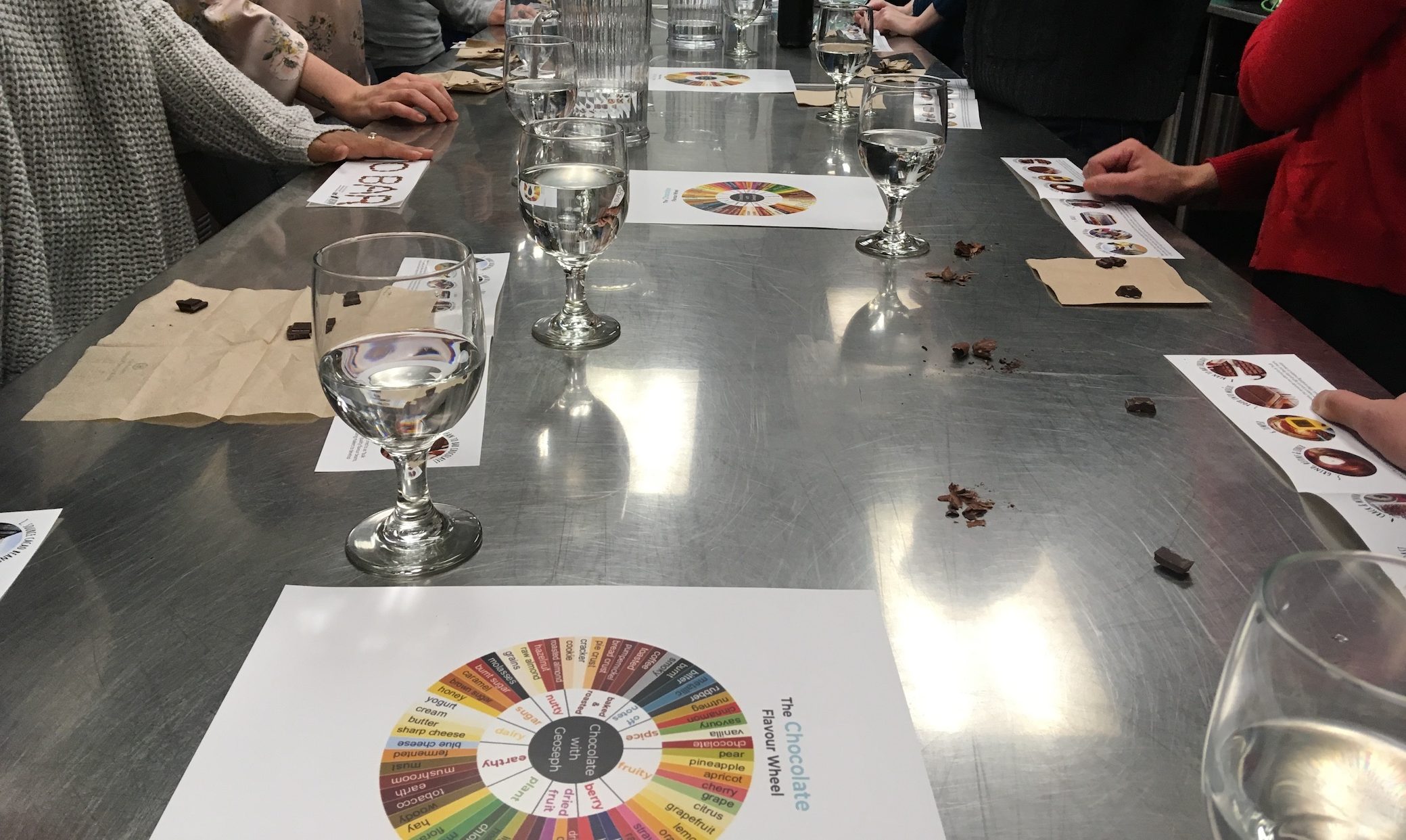The image captures a stainless steel table, marked with scratches, surrounded by approximately eight to ten people, mostly middle-aged to older adults, whose torsos and hands are visible. The participants are engaged in a chocolate tasting session, with the central focus on colorful printed sheets titled "The Chocolate Flavor Wheel." These wheels resemble a "Wheel of Fortune" with multicolored segments labeled with different chocolate flavors such as vanilla, nutmeg, fruity, spice, berry, and earthy. Scattered across the table are small pieces of what appears to be pure cacao chocolate on brown paper napkins. Additionally, there are clear goblets that likely contain water. The table also has some leaf-like debris, adding a tactile element to the scene. The participants seem to be flipping through rectangular catalogs, possibly exploring various chocolate flavors, all under bright lighting that highlights the table's silver sheen.